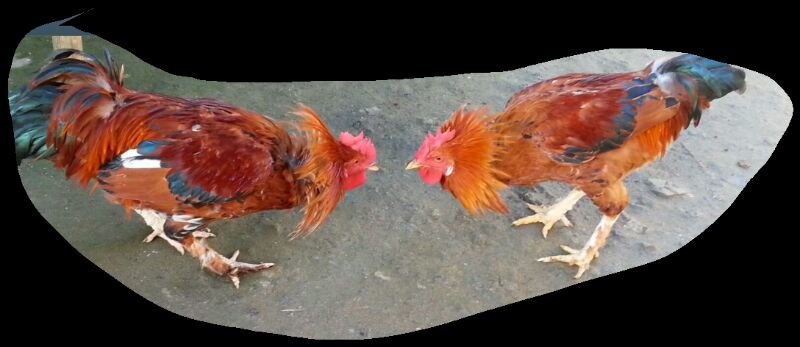The image depicts two colorful male roosters intensely staring at each other, their faces just inches apart. They stand on what appears to be a muddy or dirty concrete surface. The roosters are positioned within a haphazardly oval-cut focal point, surrounded by a blacked-out background. Both roosters feature vibrant plumage: the rooster on the right has a pink head, a brown neck down to its chest, brown feathers accented with blue on its wings, and white feet. The rooster on the left similarly has a pink face and brown neck, but its feathers are fuller, with more pronounced blue hues, particularly on its wings and tail. The feathers around their necks are fanned out, and despite their close proximity and intense posture, they seem to be sizing each other up rather than actively fighting.